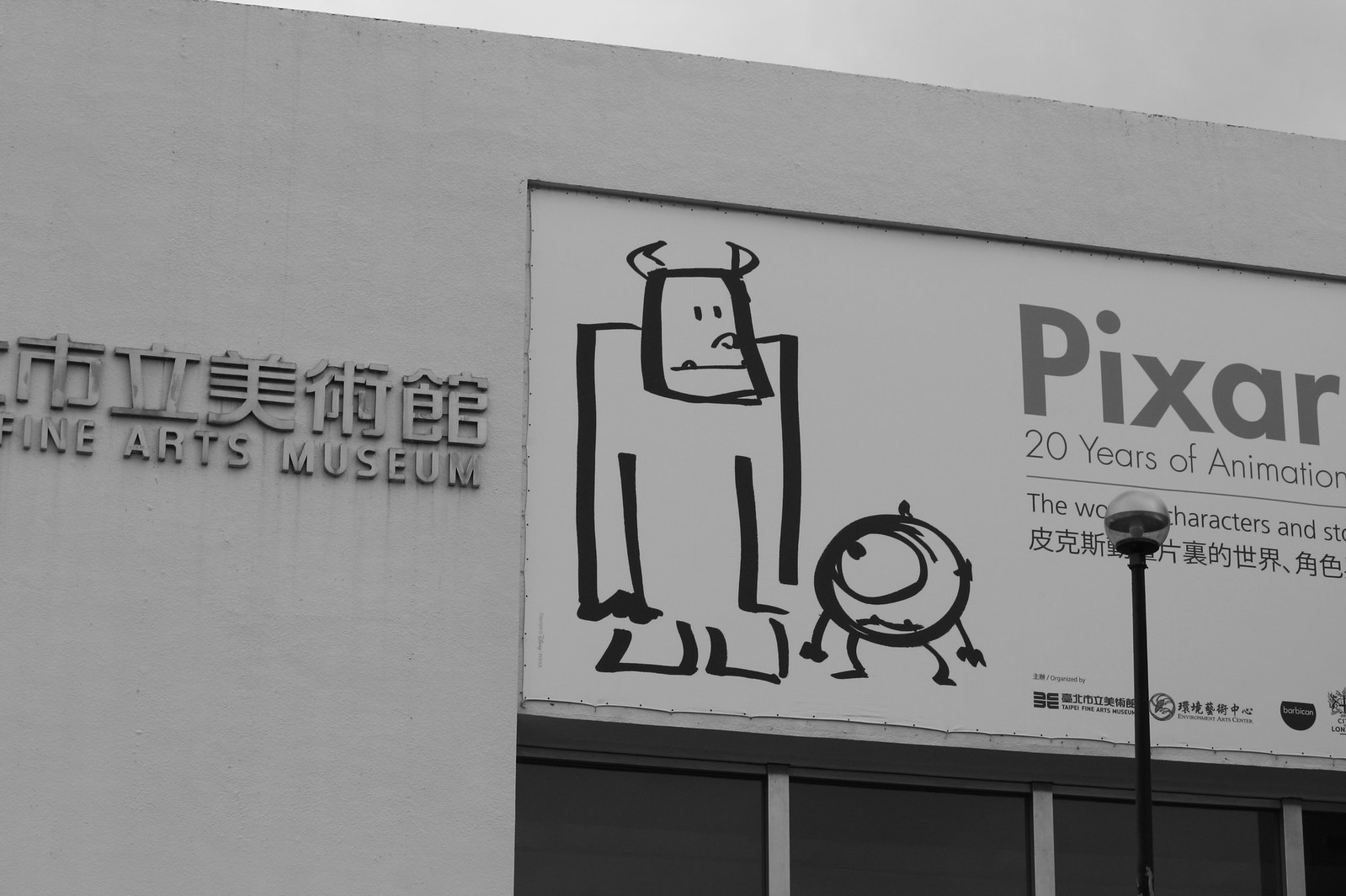The image depicts an exterior corner view of the Taipei Fine Arts Museum in Taiwan, featuring a plain white wall with a large banner sign pinned to the front. The banner advertises a special exhibition celebrating "20 Years of Animation by Pixar." The sign includes a minimalistic, marker-drawn illustration of two iconic Pixar characters: Sully, a square monster with horns and a funny face, and Mike Wazowski, a little eyeball monster, both from the "Monsters, Inc." movie. In front of the building, there is a prominent black lamp pole topped with a spherical lamp. The banner also displays text in traditional Chinese and English, identifying the venue as a municipal gallery and listing several sponsors' logos below.